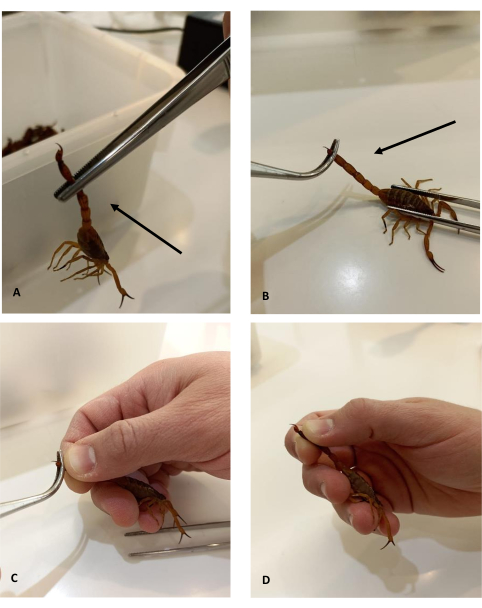The image is a vertically-oriented rectangular photo that contains four distinct subimages, arranged in a 2x2 grid with white borders separating them. Each subimage, labeled A, B, C, and D, showcases detailed interactions with a small brown scorpion. 

In the top-left image (A), the scorpion is suspended, being held by the tail with a pair of tweezers coming from the right side. The scorpion dangles with its head down, its pincers reaching out and legs hanging below. A black arrow points towards the tail, emphasizing this part of the scorpion. 

The top-right image (B) presents the scorpion lying flat on a plain white surface, which might be a bathroom or bathtub. The tweezers, silver and curved, come from the left side, still gripping the scorpion's tail. Here too, a black arrow highlights the tail.

In the bottom-left image (C), a hand appears from the right, holding the scorpion by the long segmented tail. Additional tweezers, coming from the left, assist in holding it, possibly for a closer examination or to clip something off its tail, perhaps the stinger.

The bottom-right image (D) shows the hand again, now clearly holding the scorpion to indicate the completion of some procedure, with the fingers and palm visible and pinching the tail.

The consistent creamy-colored background suggests that these images might have been taken in a controlled environment like a lab, emphasizing the procedural steps involved in handling the scorpion, possibly for study or a specific task.